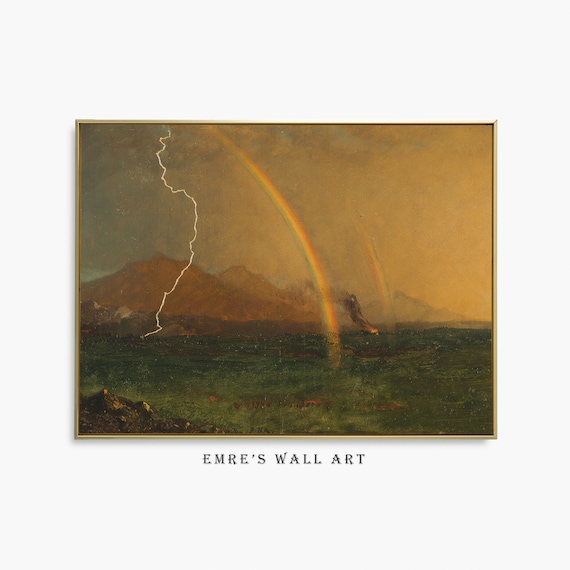The photograph captures a painting displayed on a white wall, framed in a thin brass metal frame. Below the painting, in small black text, reads "Emery's Wall Art." The painting itself is a vivid and intricate depiction of a stormy scene over a body of water. In the center, a radiant rainbow arches up towards the sky. Adjacent to this, on the left, a striking white bolt of lightning pierces downward, while on the right, flames dance on the water's surface, sending up curling tendrils of smoke. A second rainbow rises to the right of these flames. In the background, a series of four mountain peaks is visible, with hues transitioning from brown to light gray, capped with greenish grounds. The dark blue sky on the left gradually shifts to a yellow hue towards the right. A rocky shore is subtly painted at the bottom left, grounding the viewer's perspective within the scene. The overall color palette is somewhat muted, lending a somber, otherworldly atmosphere to the composition.